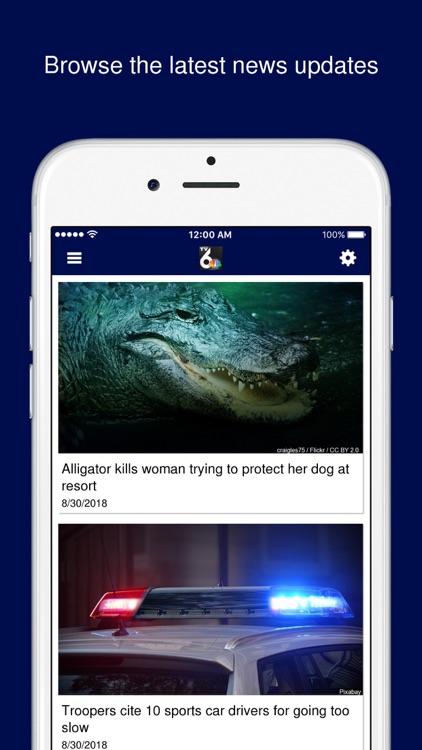The image features a phone interface set against a purple background. At the top of the phone's screen, the words "Browse the latest news updates" are displayed in white text. In the upper portion of the screen, there is a status bar with five white dots, an indication of full battery at 100%, the time displayed as 12:00 a.m., and three horizontal white lines.

Beneath the status bar, the first news headline reads, "Alligator kills woman trying to protect her dog at resort," dated 08/30/2018. This headline is accompanied by an image of an alligator. Below this, a second news story states, "Troopers cite 10 sports car drivers for going too slow," also dated 08/30/2018, and includes an image of a police car.

Both news snippets are surrounded by a thin purple border within the white phone graphic, effectively integrating the news updates within the phone interface on the purple background.